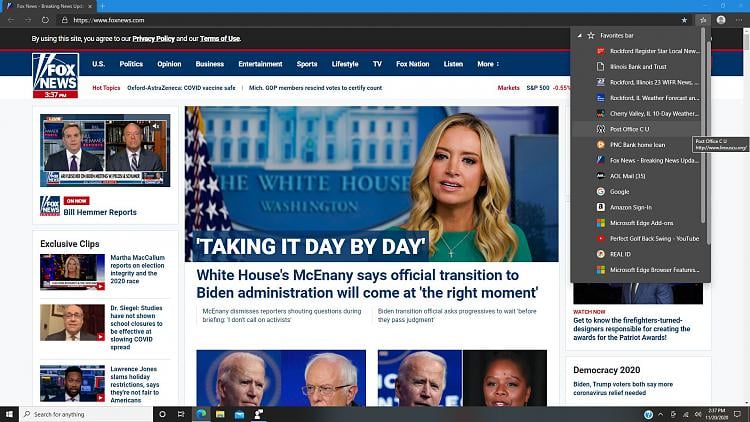This is a detailed description of a horizontal rectangular image that appears to be a screenshot from the Fox News website. 

In the upper left corner of the image, the Fox News logo is prominently displayed. It features "Fox" in white block bold lettering, right-justified, with "News" underneath it. White marks stretch diagonally from the lower left corner to the left edge at the top. A red rectangular area at the bottom edge displays the time in white.

Just above this is a navy blue horizontal rectangular bar with categories listed in white font: U.S., Politics, Opinion, Business, Entertainment, Sports, Lifestyle, TV, Fox Nation, Listen, and More.

On the left-hand side, two men are shown side by side in vertical images, though the text beneath them is unreadable. Below these images, the Fox News logo appears with "Bill Hemmer Reports" in white text. Under this, "Executive Clips" is written in black, accompanied by three horizontal rectangular areas with play buttons and different text descriptions on the right.

The central portion of the page is dominated by a large horizontal rectangular image. At the center against a light blue background, a woman appears on the right with the phrase "TAKING IT DAY BY DAY" in bold white capital letters. Beneath that, in navy blue font, it reads "White House's McEnany says official transition to Biden administration will come at the right moment."

On the right-hand side, covering part of the main image and text, there is a menu bar. This bar starts with a "Favorites" section against a light black background with white text. Each item in this menu has a corresponding logo or icon to its left.